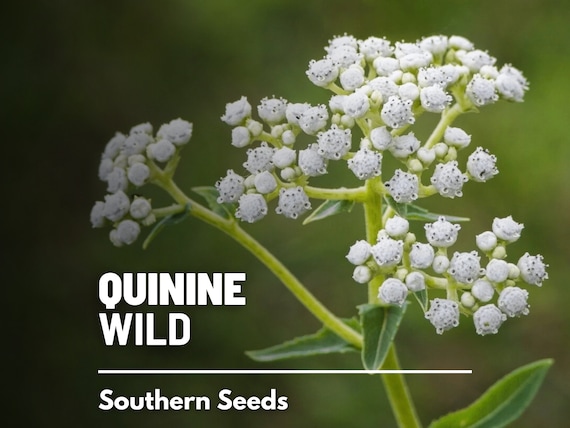The image displays a detailed photograph of a plant identified as "Quinine Wild" in prominent white, all-caps text located in the bottom left corner. Beneath this name, separated by a white line, the text "Southern Seeds" is printed in a smaller font, with only the first letters capitalized. The plant itself is shown prominently on the right side of the image. It features several light green stalks adorned with long, green, oval-shaped leaves. Atop these stalks are numerous small, circular clusters of white flowers with distinct small white dots or patterns, resembling miniature cotton balls or popcorn. The background of the image is predominantly green, with some darker, out-of-focus areas on the left, providing a contrast that accentuates the plant.